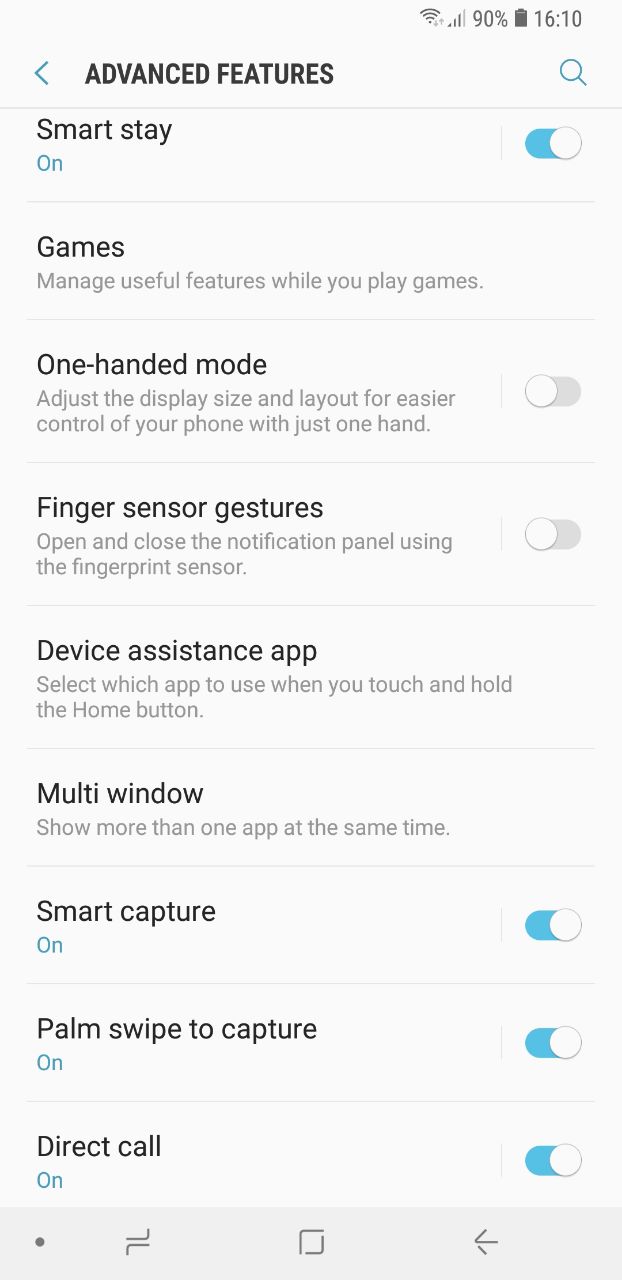This is a highly detailed screenshot of the "Advanced Features" settings on an Android mobile device. At the very top, the HUD displays a battery level of 90% and the time as 16:10. Directly below the HUD, the settings section header "Advanced Features" is indicated, accompanied by a search icon on the right for easy navigation.

The list of settings options is as follows:

1. **Smart Stay**: This feature is turned on. It uses the front camera to detect when you are looking at the screen, keeping it on while you are viewing it.
   
2. **Games**: This option allows users to manage useful features while playing games.
   
3. **One-handed mode**: Adjusts the display size and layout for easier control with one hand. This feature is currently turned off.
   
4. **Finger Sensor Gestures**: Allows opening and closing the notification panel using the fingerprint sensor. This feature is also turned off.
   
5. **Device Assistant App**: Lets you select which app to use when you touch and hold the home button.
   
6. **Multi-Window**: Shows more than one app at the same time, facilitating multitasking.

7. **Smart Capture**: This feature is enabled. It allows users to capture screenshots with extended functionalities like scrolling capture.
   
8. **Palm Swipe to Capture**: This gesture-based feature to take screenshots is enabled.
   
9. **Direct Call**: This feature is turned on. It allows the device to make a call by simply lifting it to your ear when viewing a contact's details or a message.

At the bottom of the screen, the three typical Android navigation buttons are visible: a tab button, a home button, and a back button.

The comprehensive nature of these settings showcases the depth of customization and usability options available on this Android device.